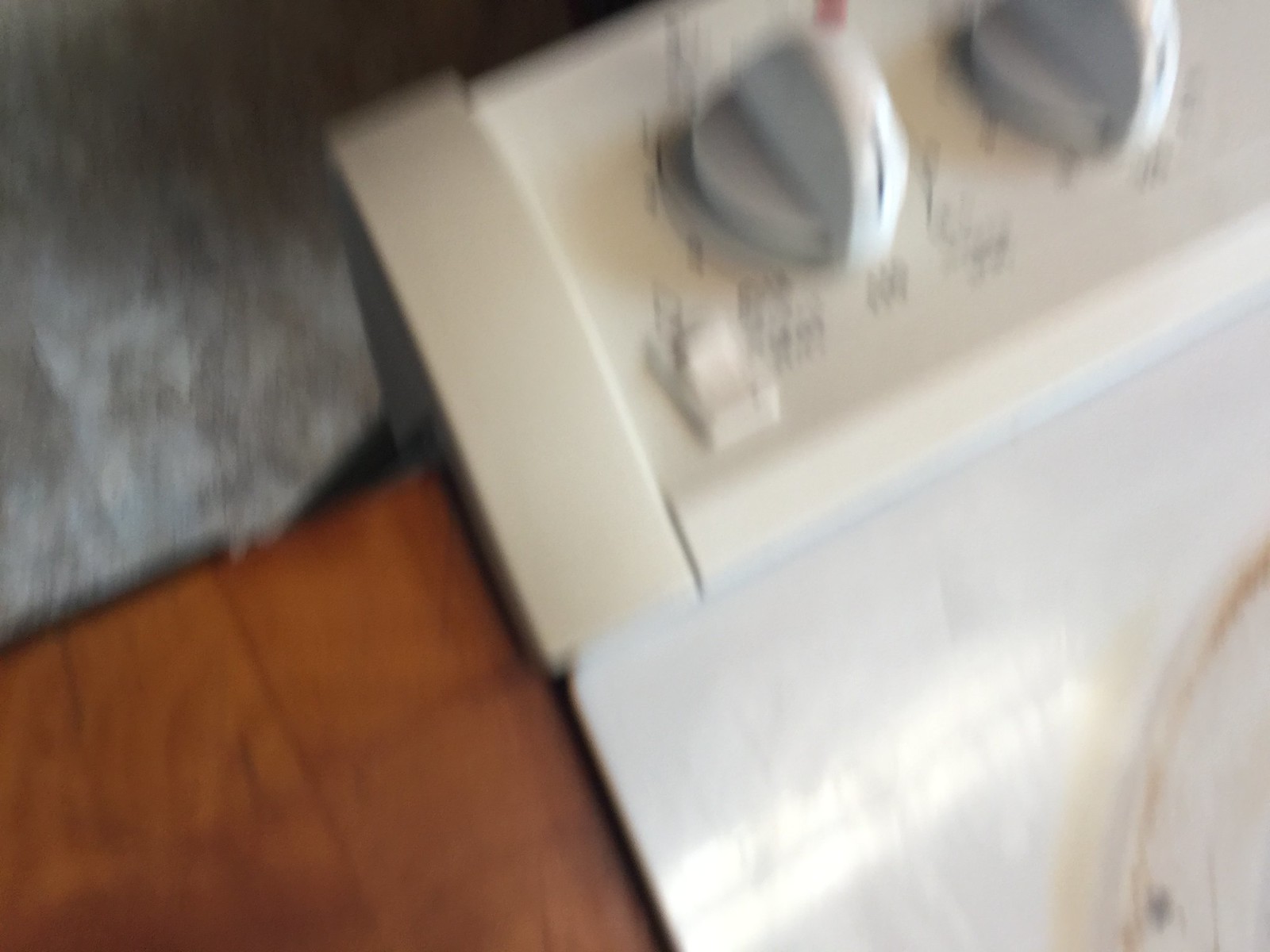The blurry photograph captures the corner of a white machine, potentially a dryer or a washing machine, partially obscured by the lack of focus. This machine features two dials on its top panel, one seemingly for setting a timer, and an adjacent switch likely serving as a start or power button. A red indicator light is visible between the two dials, possibly signifying an on/off status. Adjacent to the white appliance is a brown wooden table. In the bottom left corner of the image, there appears to be a foot with a sock, suggesting that someone is standing near the machine, likely in a kitchen or laundry area. In the background, there is a hint of a gray or light-gray carpet. The appliance also shows a brown ring around what looks to be the door, which seems to be open in this blurry and indistinct photo.